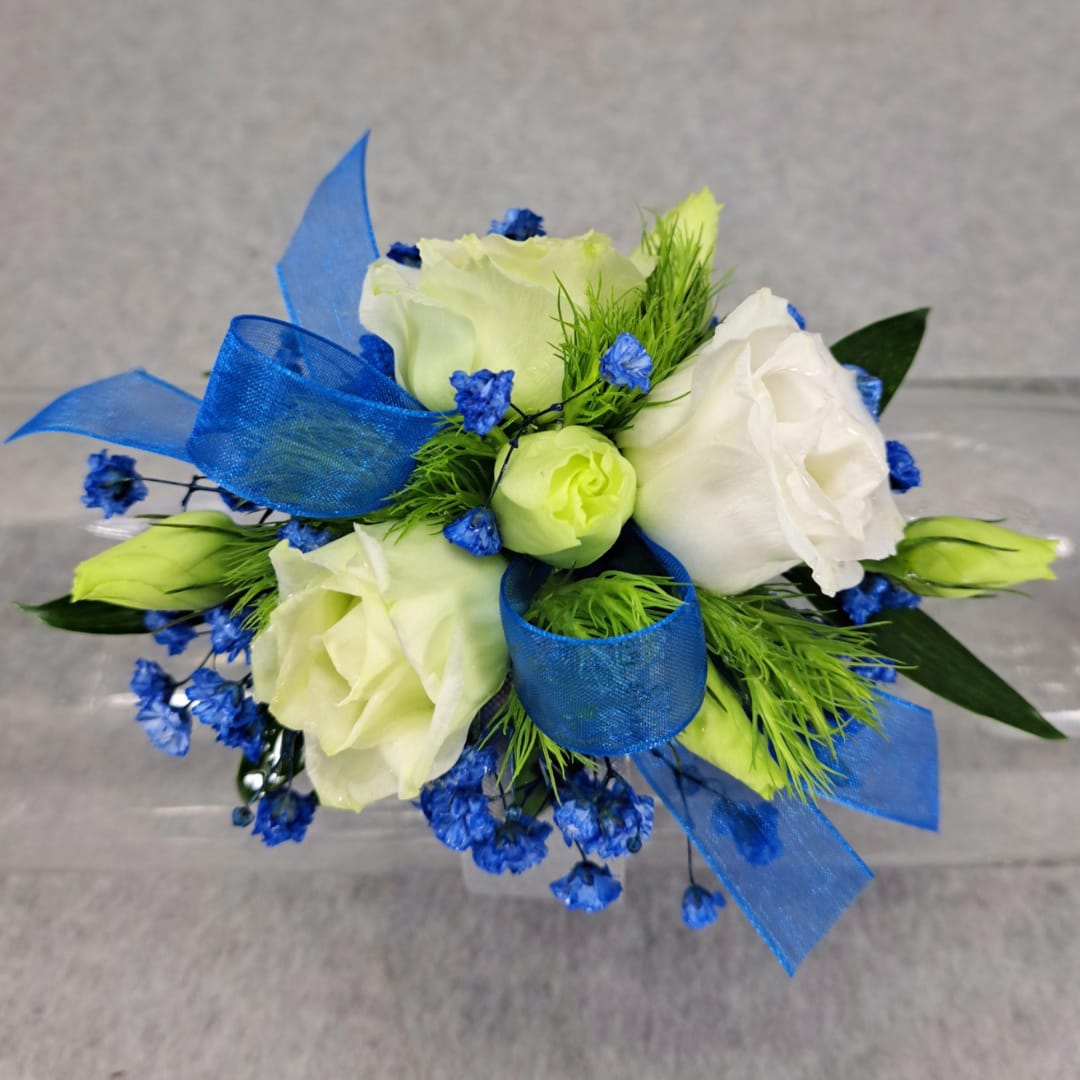This detailed photograph captures a corsage-style bouquet of flowers, showcased against a speckled gray background, possibly resembling carpet. The arrangement is viewed from above in a bird's-eye perspective, highlighting both the flowers and the intricate details. Dominating the bouquet is a blue see-through ribbon tied into a bow at the center, with its ends gracefully extending toward the top and bottom right corner.

At the heart of the bouquet are several flowers, including two yellow roses, one white rose, and a greenish bud that is yet to bloom, nestled centrally. Interspersed among these are tiny blue flowers, similar to baby's breath, adding a delicate touch. The bouquet also features dark green leaves and other light green plants resembling grass, providing a contrasting texture and additional richness to the overall composition. Draping the arrangement is a wide cellophane band running horizontally, blending seamlessly with the gray background, which transitions from a solid gray at the top to a line in the middle, and then back to a solid gray at the bottom. This subtle backdrop highlights the flowers and their colorful bow, making them the focal point of this beautifully arranged photograph.